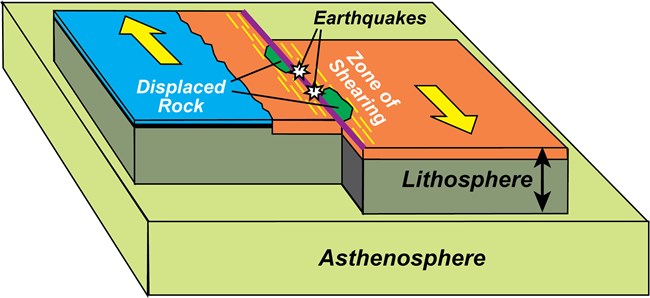The image is a 3D graphical representation depicting geological layers. At the base, there is a sizable yellow block labeled "ASTHENOSPHERE" in black text, clearly visible at the front of the block. The block is slightly tilted to the right, allowing viewers to see both the front face and the right side of this foundational layer. Resting atop the yellow base are two smaller blocks. The block on the right is labeled "LITHOSPHERE." Additionally, there is a label marked "Earthquakes" with two arrows pointing downward to the meeting line between the two top blocks, indicating the area where tectonic interactions that cause earthquakes occur.